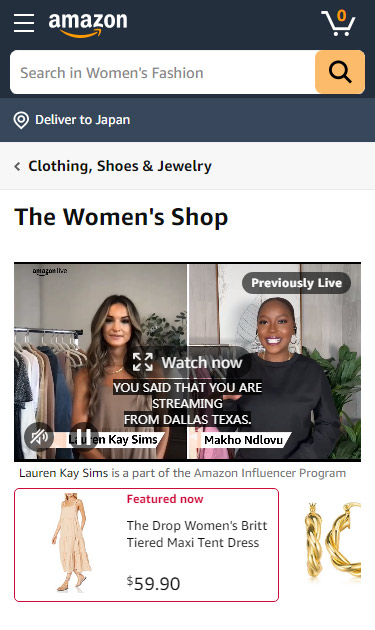This image is a screenshot of an Amazon web page displayed on a smartphone, evident from its long and narrow format. At the top of the page, the Amazon logo is prominently displayed, composed of three horizontal lines followed by the word "Amazon" accompanied by its iconic orange curved arrow. To the right of the logo, there is a shopping cart icon with a ‘0’, indicating an empty cart.

Beneath the logo, a search bar is visible, prompting users to "Search in Women's Fashion." Adjacent to the search bar, there's a pin location icon indicating that the delivery is set to Japan. Just below this, there's a left-facing arrow beside the category label, "Clothing, Shoes, and Jewelry."

The main heading "Women's Shop" is prominently displayed, signifying the section of the website. Underneath this heading are two side-by-side photos. The left photo features a white woman standing in what appears to be a store, while the right photo shows a Black woman standing possibly in an office setting. Both images are overlaid with a small black oval banner at the top labeled "Previously Live."

In the center of these images, bold text urges viewers to "Watch now." It also states that the streaming location is from Dallas, Texas, with names appearing in front of each woman. Additionally, a sound icon with a line through it indicates that the audio is muted.

Below these images, text informs readers that "Lauren K. Sims is part of the Amazon Influencer Program." Further down, a square with a red border highlights a woman modeling a dress with the caption, "Featured Now." The item is "The Drop Women's Brit Tiered Maxi Tint Dress," priced at $59.90. To the side of this image, a pair of gold hoop earrings, described as braided, are also featured.